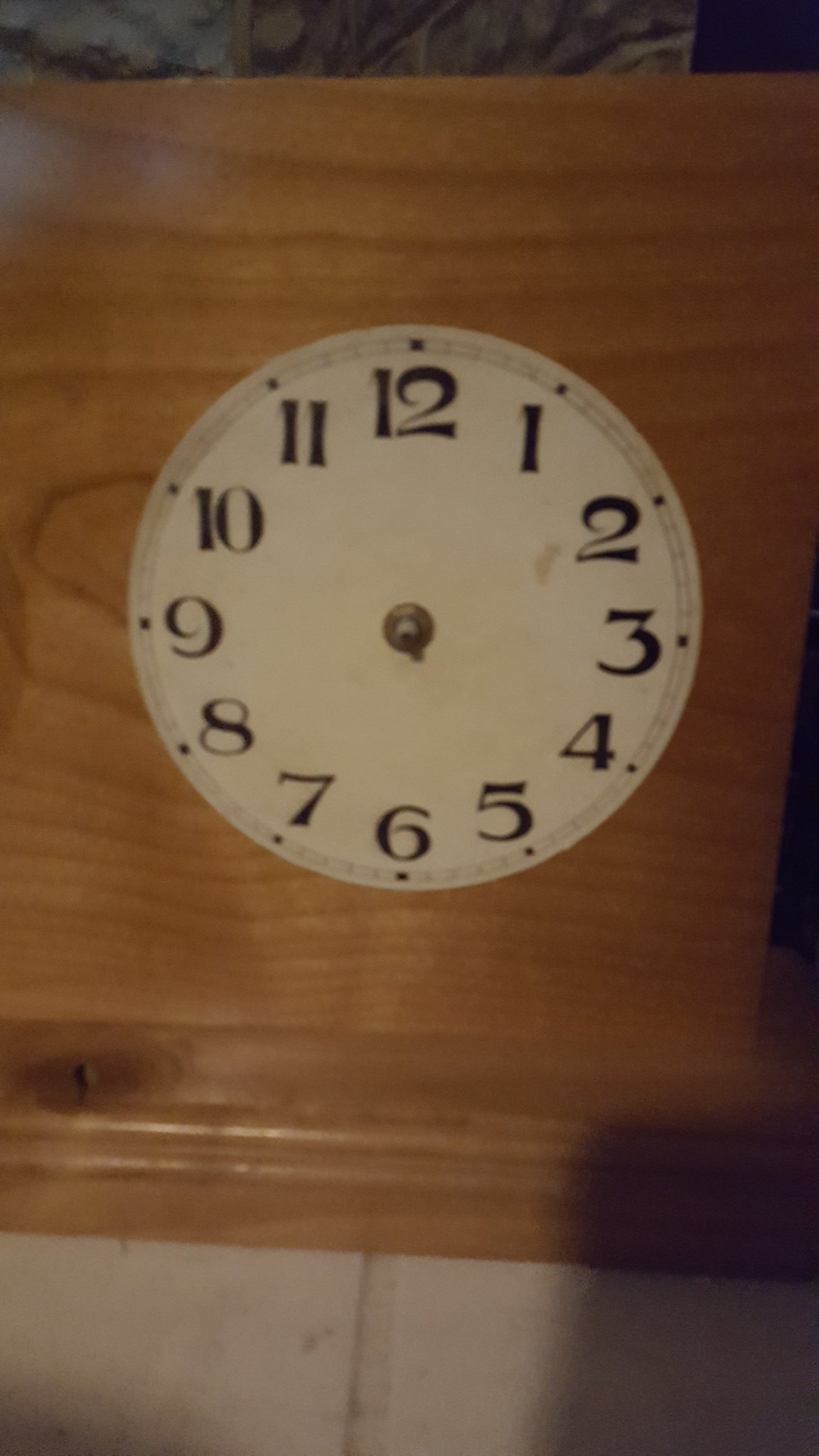This image depicts a wooden clock under repair, displayed on a light wood base with distinctive grain patterns, including a visible pine knot in the bottom left corner. The clock itself consists of a circular white face, which is notably devoid of hands, revealing only a central metal knob with a line extending towards the number 5, hinting at its previous operational state. Surrounding the face, the numbers 1 through 12 are prominently marked, with small black squares positioned above each number and alternating gray and white squares between them. The scene is set on a tile floor with pronounced grout lines, indicating the sizable tiles. In the upper part of the photo, there are two reflections of light in the top left corner of the clock, adding brightness to the otherwise softly lit setting. A faint background is visible at the top of the photo, yet it remains out of focus, while the photographer's shadow can be noticed at the bottom right.